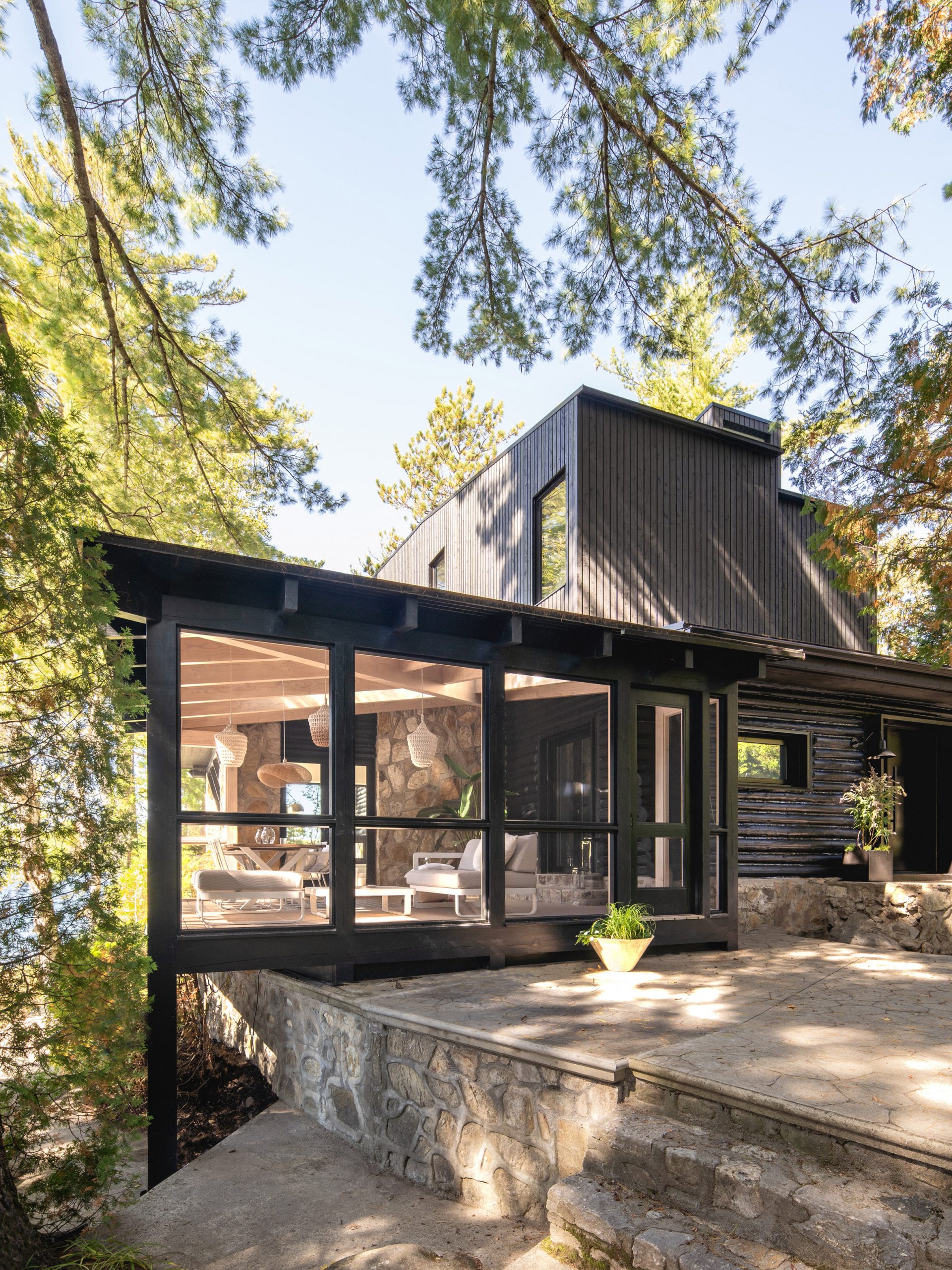This daytime photograph captures the elegant exterior of a well-designed, modern two-story house nestled in a thickly forested area. At the very top of the image, a clear blue sky fades to a whitish hue towards the horizon. Tall trees frame the scene, their green branches extending over the roof and partially shading the house.

The house itself features a distinct dark color palette, predominantly composed of black wooden slats and dark brown and gray stone elements. A prominent section of the house, seemingly a lounge area or enclosed patio, is made entirely of glass walls, allowing a clear view into a modern living space adorned with white sofa chairs and other contemporary furniture.

On the right side of the house, the structure is distinctly two stories tall, with large rectangular windows adorning both levels. Below these windows, a cobblestone path leads up to stone steps at the front right of the image, contributing to the stately entrance.

Additionally, two potted plants are positioned near the center and slightly to the left of the house, adding a touch of greenery to the immediate surroundings. The overall scene is highlighted by the vibrant green of the trees and the bright sunlight filtering through, casting light and shadow across the house's exterior.